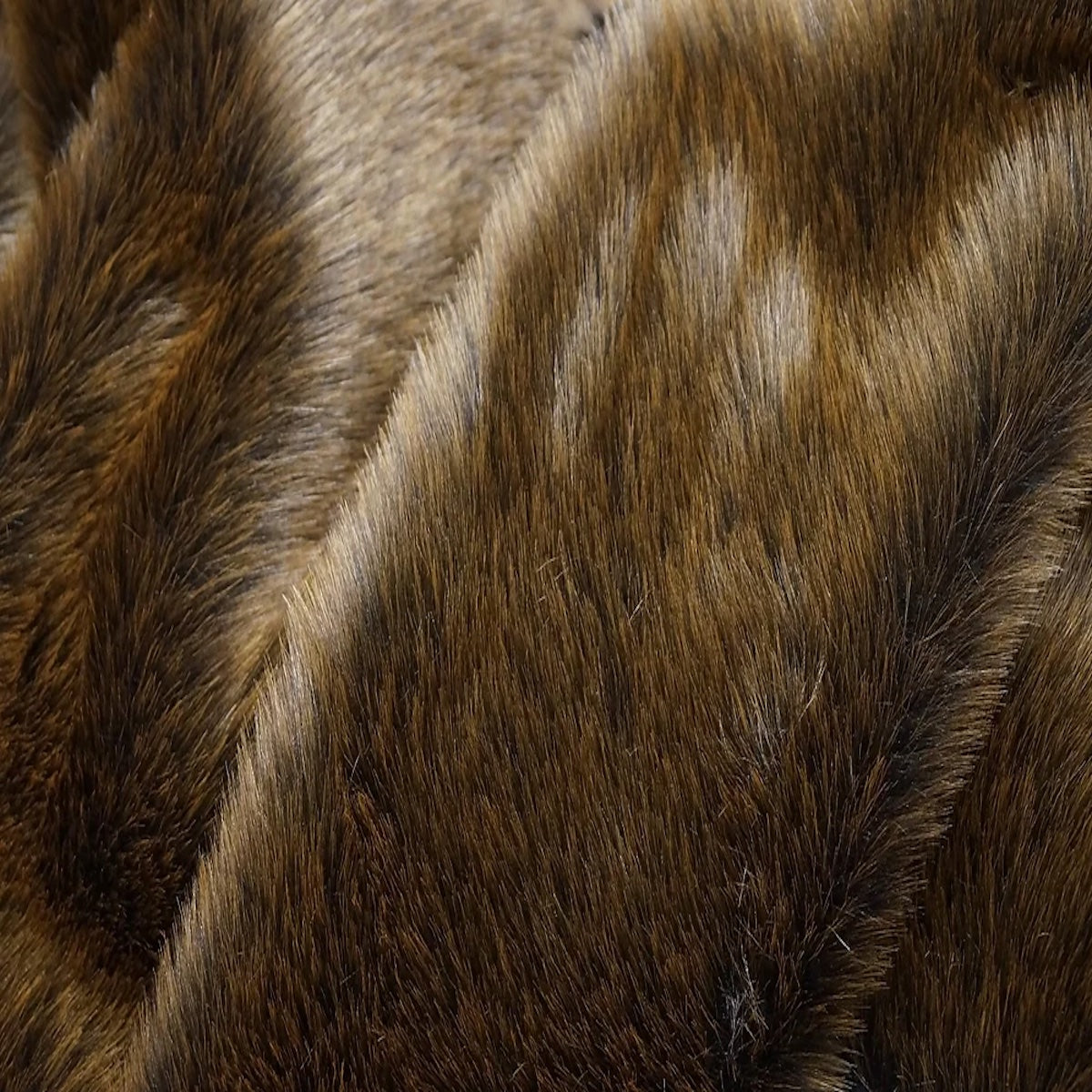This image captures a highly detailed, close-up view of an animal's fur, possibly a cowhide or bearhide, featuring a rich mixture of dark brown, beige, and tan colors. The fur appears exceptionally shiny and healthy, reflecting light in a way that highlights the bristles, which are mostly oriented upwards. Some trimmings of hair rest on the fur itself, adding to the texture. The photograph focuses solely on the fur, omitting any visible eyes, body, or limbs of the animal, and it's taken from a top-down perspective. The fine individual hairs are distinctly visible, showcasing the fur's varied shading and intricate details.